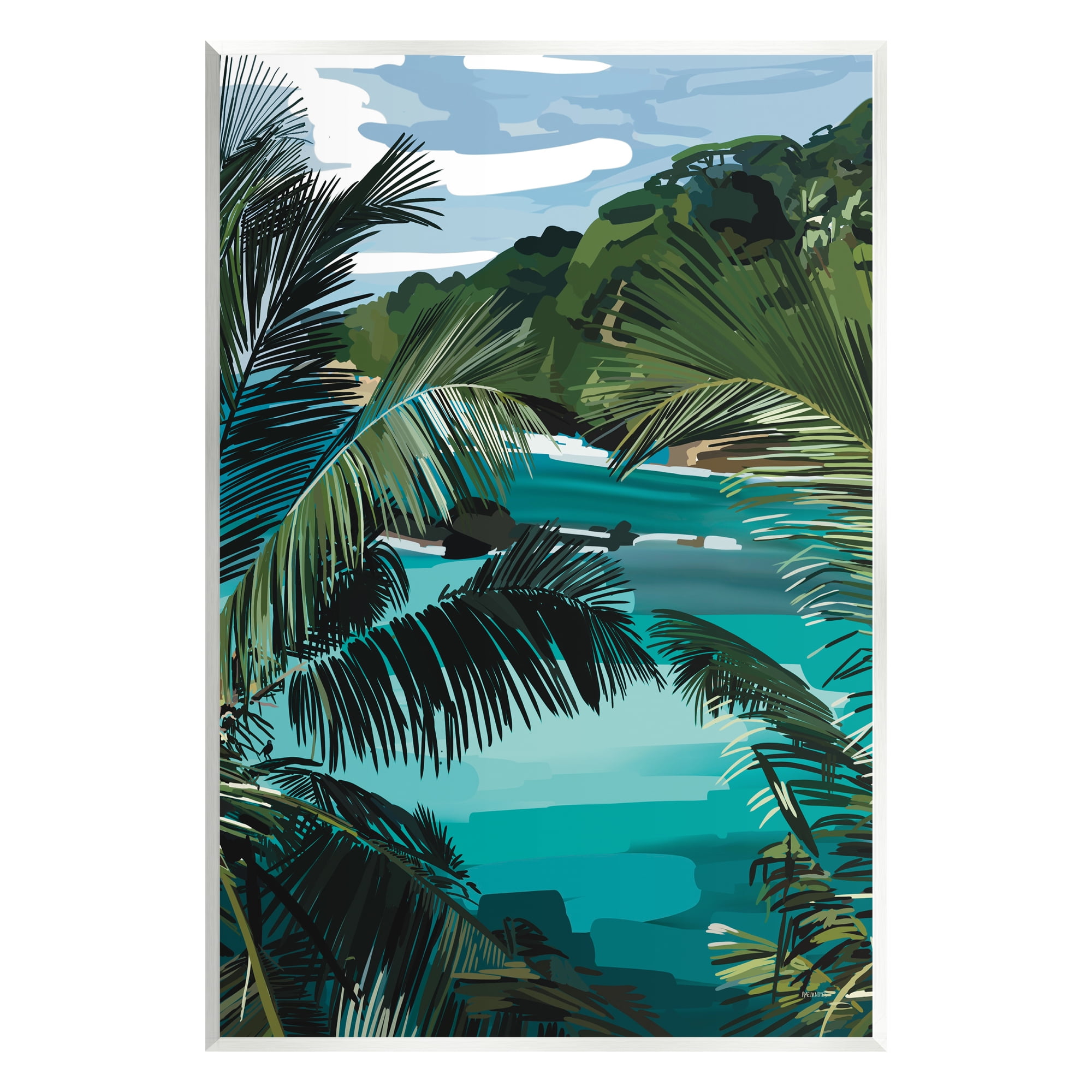This is a blocky, impressionistic painting capturing a serene tropical shoreside scene. The composition is framed with a white border that accentuates its vivid colors and textures. At the top, a deep blue and light blue sky is dotted with whispering white clouds, creating a tranquil atmosphere. In the top right, blocky smudges of green—in shades ranging from olive to lime—descend towards the center left, suggesting lush vegetation or a forested area. Below this greenery, a teal, aqua, and light blue body of water stretches across the scene, with white stripes marking the shoreline where it meets the dense forest.

Framing the painting are palm fronds, which extend from the left, right, and bottom borders into the center. These fronds vary in color and shade, with some appearing dark and silhouetted, especially on the left and bottom left, and others displaying hues of olive green to sand green on the left, right, and bottom right. The fronds partially obscure the view, lending a sense of peeking out from a hidden vantage point. This vantage point reveals more details of the tropical setting: bluish-greenish water with a hint of crashing waves, and a tranquil, almost untouched ambiance. The overall impression is one of peacefulness and relaxation, providing a snapshot of a serene, hidden paradise.